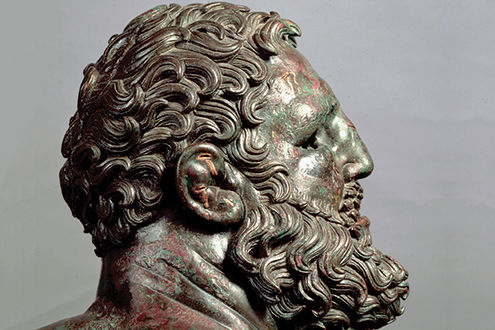The image is a detailed photograph of a bronze statue, focusing on the head in a side profile. The statue, likely of Greek or Roman origin, depicts a male figure with strong facial features. His eyes are closed, and he has a distinct cauliflower ear, suggesting he may have been a wrestler. The man's hair is abundantly curly, complemented by a long, wavy beard, both intricately textured with swirly waves. The statue exhibits a bronze green patina with red highlights, giving depth to the hair and beard. The background is entirely grey, further emphasizing the aged and somewhat rusted appearance of the statue's neck, reflecting its historical significance.